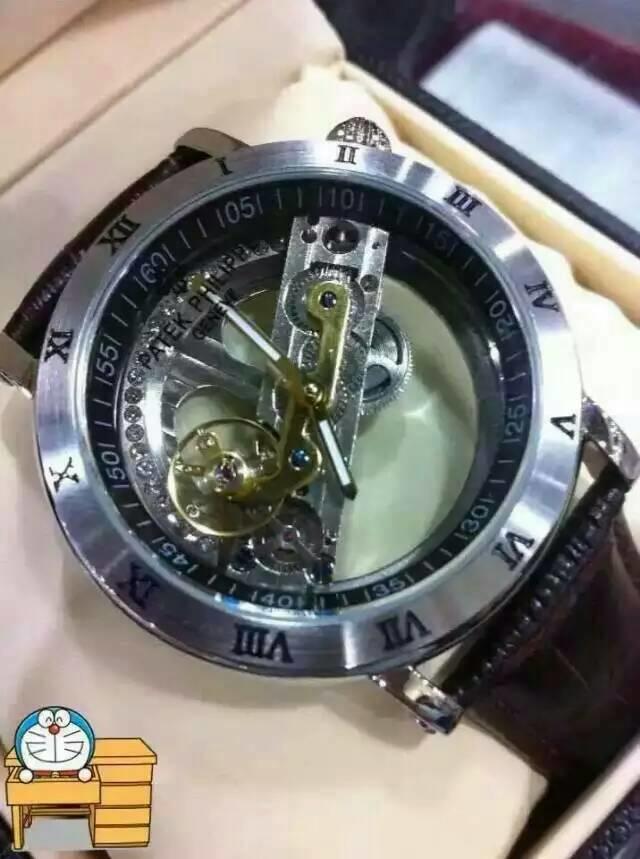This image features a meticulously crafted silver wristwatch with a round face. The dial prominently displays elegant Roman numeral hour markers, exuding a timeless classic aesthetic. The centerpiece of the watch’s design—a transparent section—reveals the intricate inner workings, highlighting the prestigious craftsmanship of Patek Philippe. The inscription "Patek Philippe Genève" is elegantly printed in black text at the center of the dial. Surrounding the inner rim of the watch are various numerical markers: 160, 105, 101, 151, 20, 25, 30, 35, 40, 45, 50, 55, and 60, arranged in a clockwise fashion. At the bottom of the watch face, an animated illustration depicts a whimsical scene of a blue character with a white base and expressive eyeballs, peeking out from the front drawer of a desk, adding a playful touch to the sophisticated timepiece.